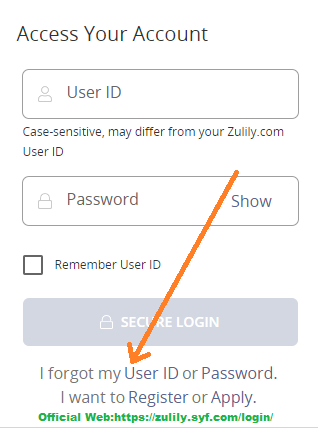The image depicts a login page featuring a largely white rectangle with most edges not visible except for the bottom, where a gray line extends the width of the form. The heading at the top reads "Access Your Account." Below, there are two input fields: the first labeled "User ID" with the note "Case-sensitive, may differ from your ZULILY.com user ID," and the second labeled "Password," accompanied by a "Show" option on the right side. 

Beneath the input fields, an unchecked checkbox is labeled "Remember User ID." Further down is a gray and white button labeled "Secure Login," followed by a "Forgot my User ID or Password" link highlighted by an orange arrow pointing downward from the "Show" button; the arrow appears slightly ragged, indicating it was added using a photo editor. 

The caption continues with the text "I want to register or apply," and below that, in green, it reads "Official web: https://ZULILY.SYF.com/login/." The dominant colors in the image are black, gray, white, orange, and green. The image appears to be full-size and does not require enlargement.